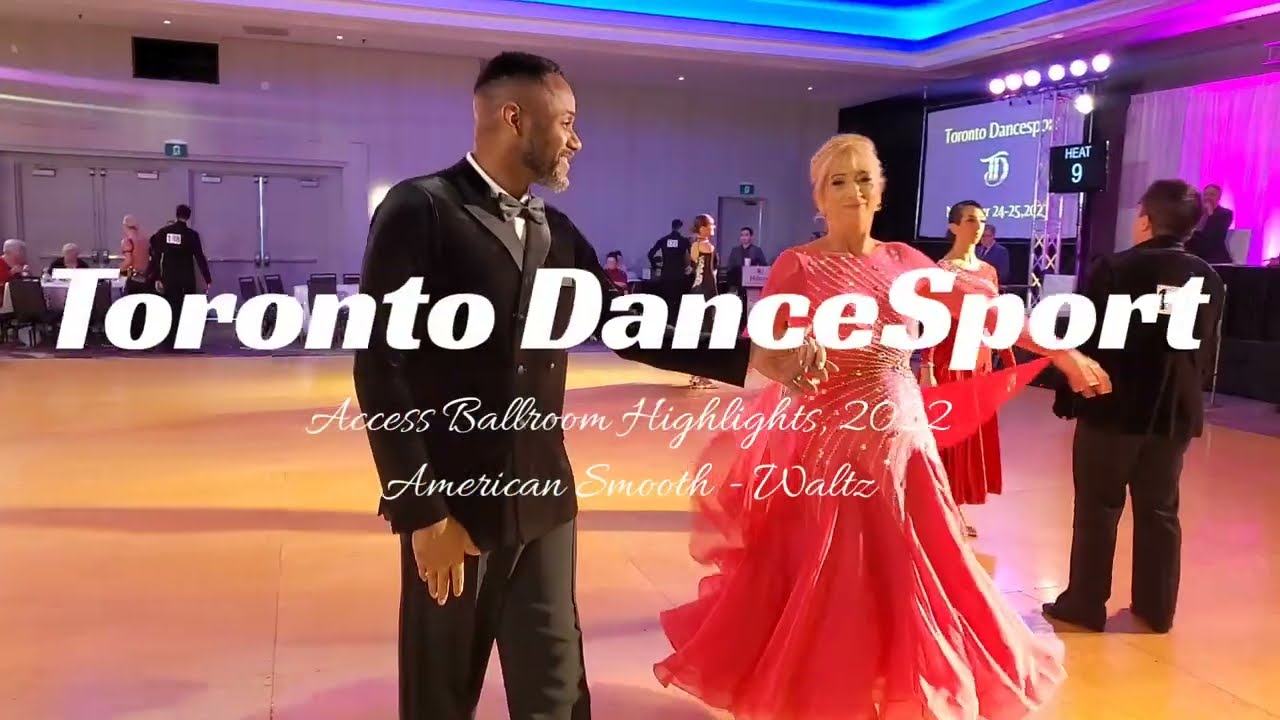The advertisement image is a vivid, indoor color photograph in landscape orientation, capturing an elegant ballroom scene adorned with various hues of purples and blues, illuminated by neon lights along the ceiling. Dominating the dance floor in the center, a graceful African-American man clad in a black tuxedo with a gray bow tie extends his hand to a blonde Caucasian woman, approximately 50 years old, who smiles up at the viewer. She elegantly wears a dark pink, sparkly gown with a full skirt that flows to the ground and a scarf attached to her wrist. The ballroom is abuzz with activity, as other figures in the background also appear to be dancing under the vibrant lighting.

In the middle of the image, bold white letters spell out "Toronto Dance Sport." Just beneath this main title, in fine cursive, the text reads "Access Ballroom Highlights 2012," with "American Smooth Waltz" written below it. On the right-hand side, a small black sign with white letters displays "HEAT9." The scene exudes a lively and sophisticated ambience, emphasizing the prominence of the dance event and the elegance of the participants.